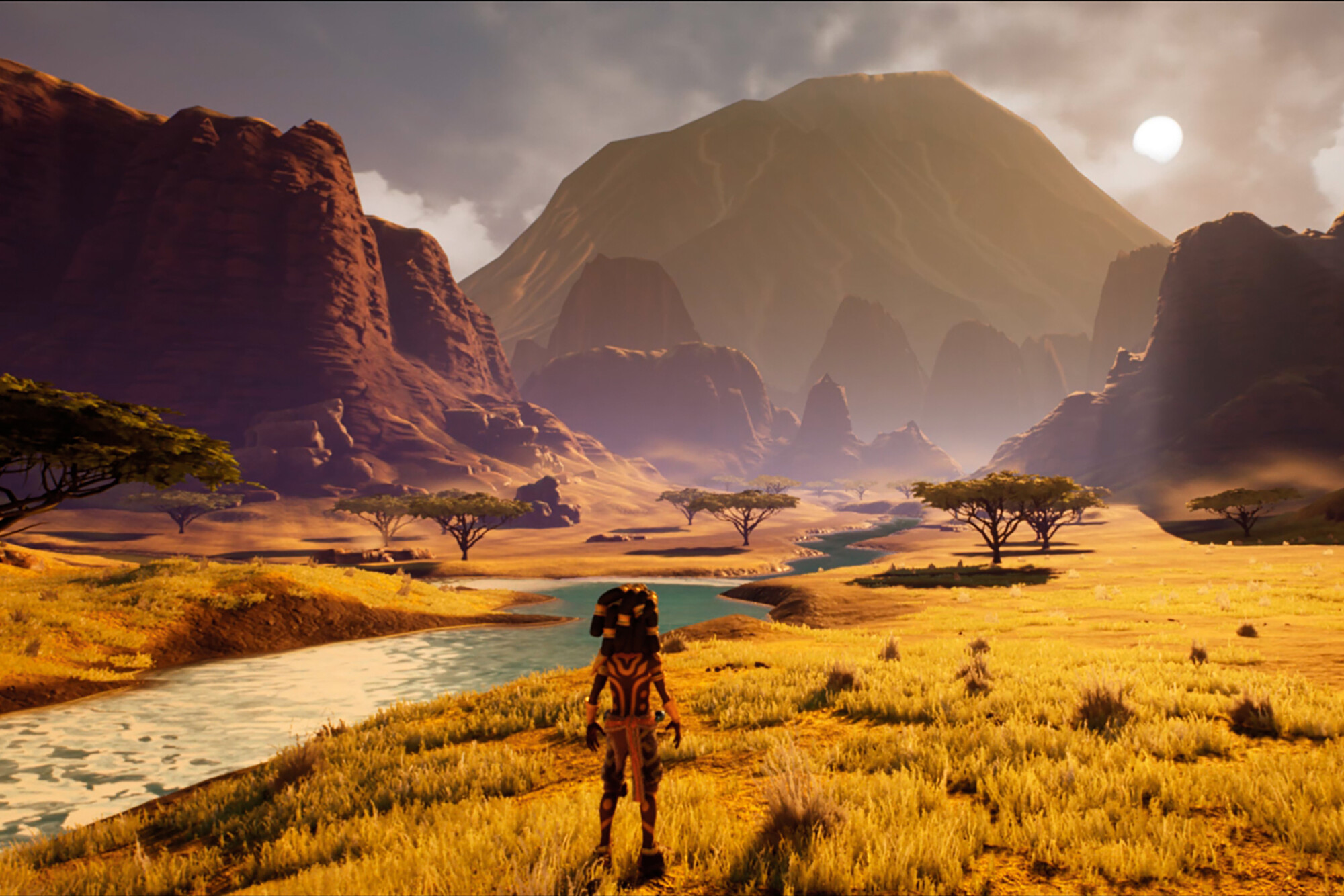The image depicts a scene reminiscent of either a video game or an animated cartoon, rendered in an ultra-realistic style. Dominating the background is a large, ominous mountain under a dark sky. To the right of the mountain, a white celestial body—possibly the sun or the moon—peeks through the smoky atmosphere.

In the valley below, two imposing cliffs flank either side; both are predominantly brown. Furthermore, the landscape transitions to a sunny section near the bottom of the image, revealing a mix of yellow and green grass interspersed with yellowed flowers.

A stream cuts through the valley, originating from the left bottom corner and meandering towards the center-right of the image. The water is primarily blue but reflects shades of yellow and white where the sunlight strikes it.

Scattered within the scene are trees with black tops and green foliage supported by brown trunks. Central to the composition is an alien-like creature or man standing at the forefront. The figure wears a black-orange head covering and an outfit consisting of an orange and black vest and pants, which blends with the earthy and contrasting tones of the landscape. The overall surreal yet highly detailed environment creates a captivating and mysterious visual narrative.